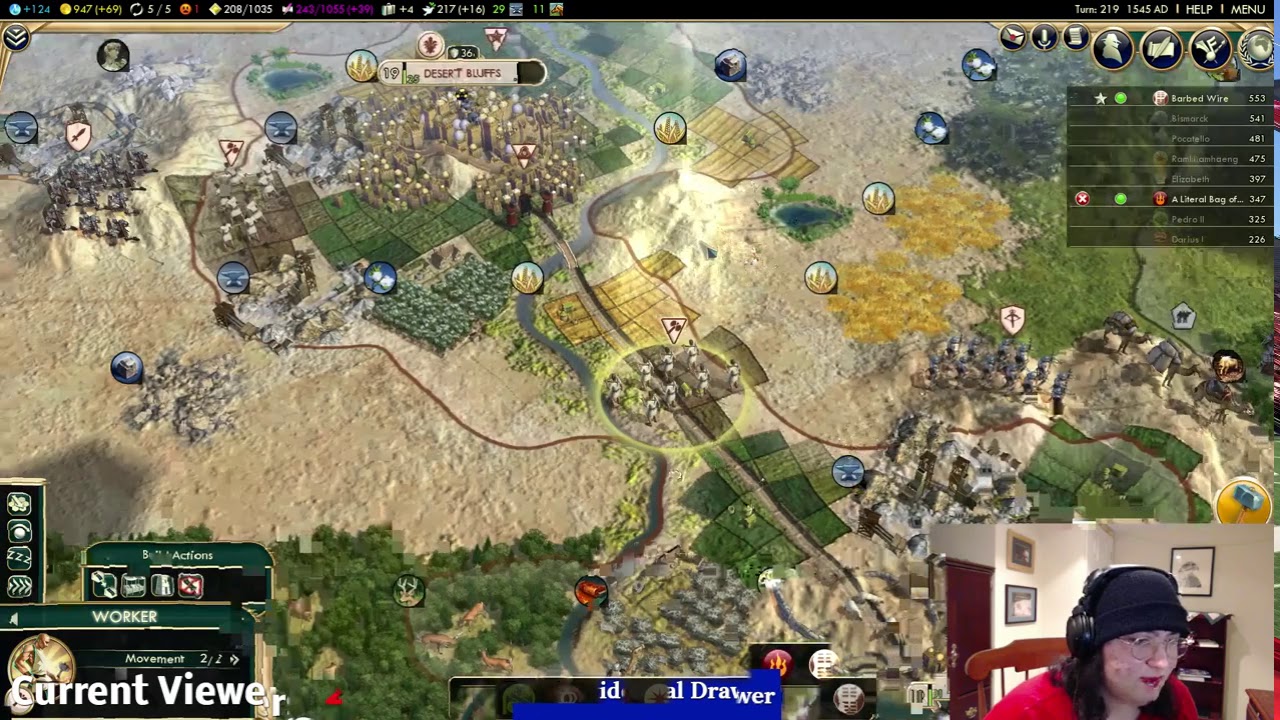The image is a detailed screenshot of a video game live stream. In the bottom right-hand corner, there's a small rectangular overlay showing the video game streamer. The streamer, who appears to be a young, possibly female individual with long hair, is wearing a black toboggan, round silver-rimmed glasses, and a pair of headphones. They have notably red lips and are seated in a brown wooden chair. Their attire includes a red shirt, and the background shows white walls adorned with pictures. The streamer is playing a real-time strategy game, with an overhead view of a landscape that resembles a field or a kingdom. In the center of the game screen, there is a noticeable green circle with figures in light-colored uniforms, possibly representing armies. Overlay text on the game screen includes "current viewer" in the bottom left corner, and partial text in the center undergoing an animation transformation, including the letters "ID... drawer." Additional graphics may indicate game elements like lives or weapons.